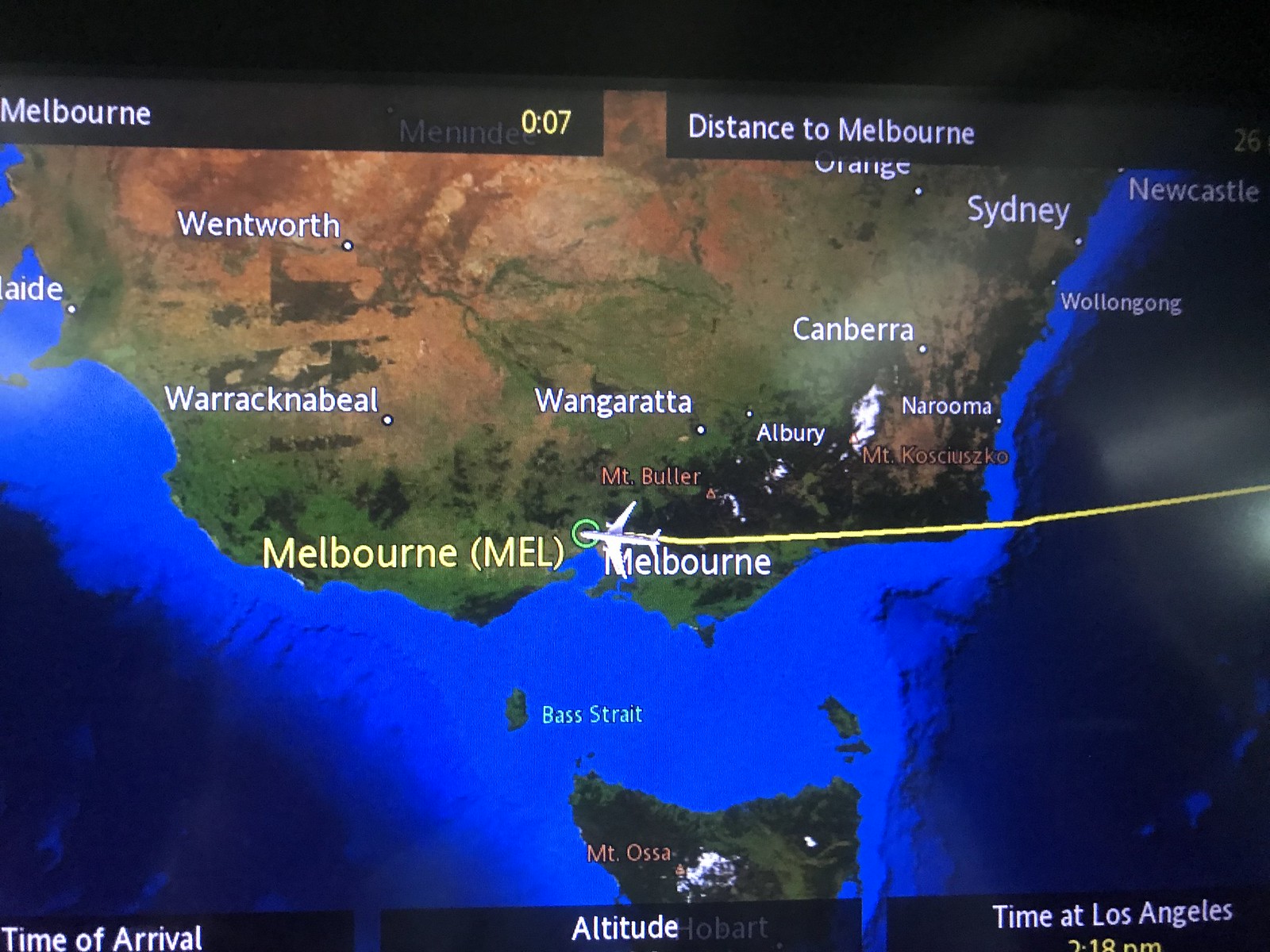The image is a photograph of a digital map displayed on a monitor, depicting the flight path of an airplane over Australia. At the top left of the screen, within a black banner, "Melbourne" is displayed in white text, followed by "0:07." Another black banner on the right side of the screen shows "distance to Melbourne." The map itself features white-labeled locations including Wentworth, Warwick Neville, Wangaratta, Canberra, Sydney, Albury, Naruma, Wollongong, Newcastle, and Melbourne, with red labels for MT.Buller and MT.Kosciuszko. A yellow line stretches across the map, indicating the airplane's flight route, accompanied by a white graphic of an airplane. Blue text at the bottom of the map names the Bass Strait, with “MT.Ossa” also marked. Additional black banners at the bottom of the screen provide flight details: "time of arrival" on the left, "altitude" in the center, and "time at Los Angeles" on the right, the latter showing a partially visible yellow timestamp, "2:18 p.m." The screen also displays varying landscapes of Australia, highlighting green areas and desert-like regions, set against a blue ocean background.